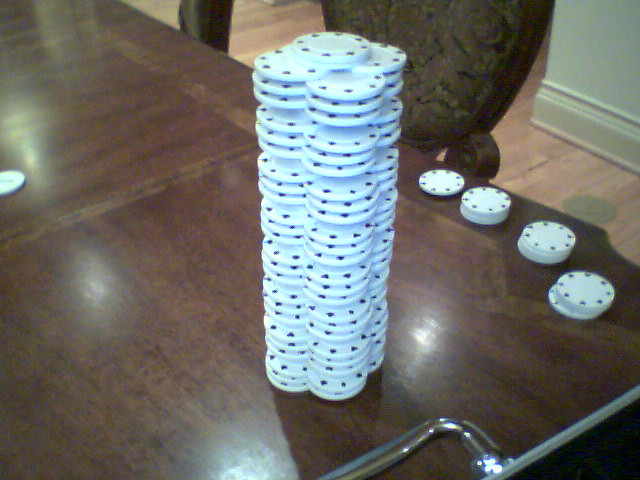The image is a color snapshot with considerable glare and focus issues. It predominantly features a dark, polished wooden table with an intricate inlaid design, which takes up most of the frame. The table has a glossy finish with an unusual clear acrylic edging on one side. Resting on the table are numerous stacks of poker chips, predominantly white with eight small black symbols—likely hearts or diamonds—around the perimeter, arranged like the numbers on a clock.

The focal point is an elaborate structure made from poker chips, consisting of four interlocking columns forming a single tall tower topped with one chip. The tower segments resemble flower petals projecting outward. Alongside the tower, there are smaller stacks of poker chips in a row, increasing in height progressively from about two to five chips. Additionally, a loose poker chip lies near the bottom right corner of the table.

In the background, at the upper right of the photo, is the back of an ornately carved oval wooden dining chair. The scene includes a glimpse of a hardwood floor, a small section of an off-white wall, and matching baseboard molding. This cozy, yet somewhat cluttered residential setting offers a casual, lived-in feel.